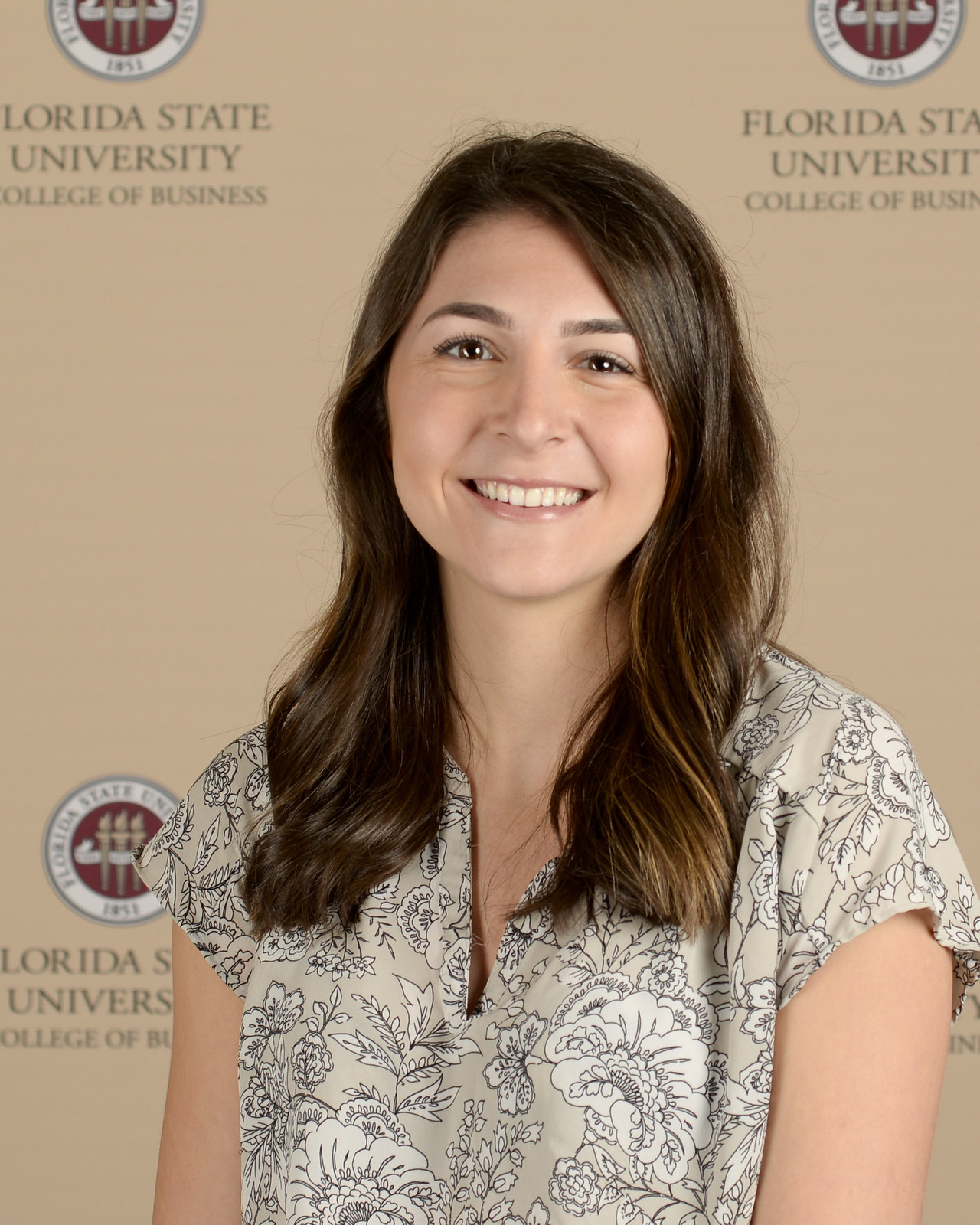This is a detailed portrait of a young Caucasian woman, likely in her early to mid-20s, with a cheerful demeanor. She is looking straight at the camera with a radiant smile, revealing her white teeth. Her brown hair, adorned with subtle blonde highlights at the tips, is styled into a slight curl and parted to the side. She also has brown eyes and is wearing a bit of red lipstick.

The woman is dressed in a short-sleeved, v-neck floral shirt, predominantly light tan or cream in color. The shirt features a pattern of white flowers and leaves outlined in black. The background of the image displays the Florida State University College of Business logo, which is repeated in all four corners. The logo has a white circular edge surrounding a smaller red circle containing three torches intertwined with a white banner that reads "1851". The text "Florida State University" appears in a larger sans-serif font, while "College of Business" is styled in a smaller sans-serif lettering beneath it. 

The overall scene sets a professional and welcoming tone, highlighting the woman's connection to Florida State University’s College of Business against a beige backdrop with the institution's emblem prominently displayed.